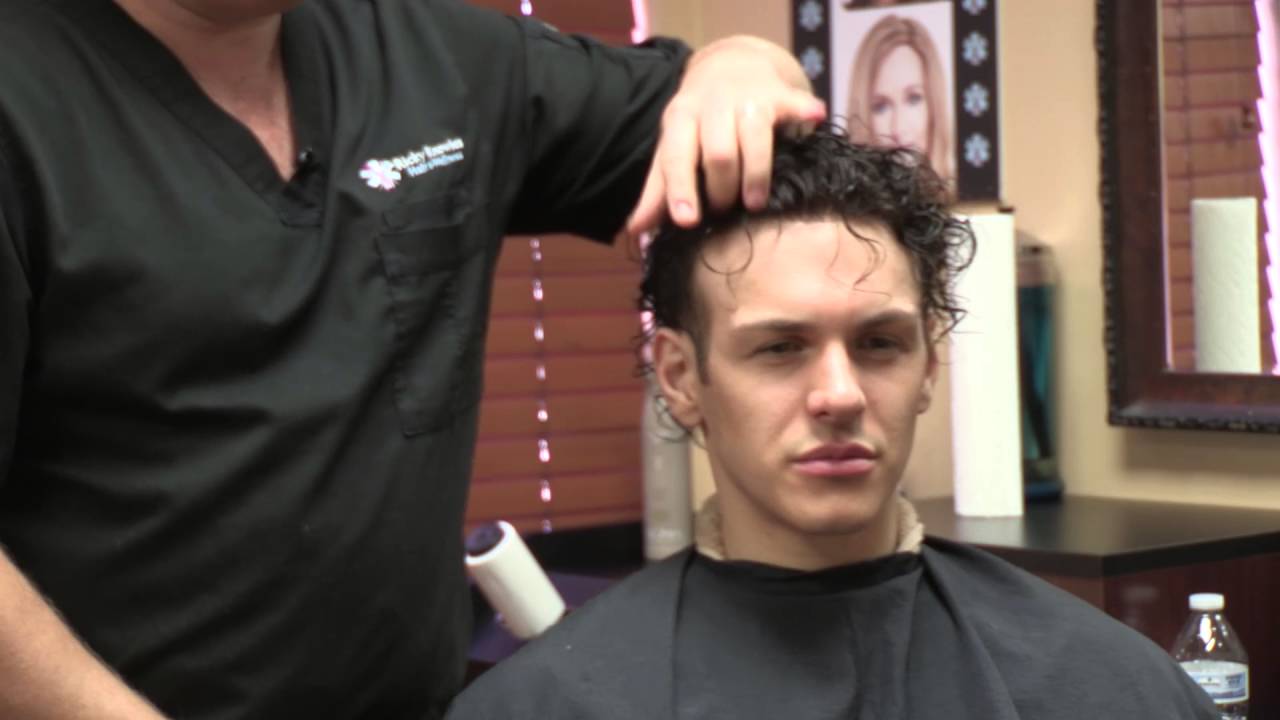In the image, a young man with dark, slightly damp and curly hair is seated, ready for a haircut. A barber, dressed in a black v-neck shirt adorned with an unreadable logo on the left side, is seen demonstrating a haircut technique. The barber's hands are attentively positioned in the client’s curls, likely planning the next steps of the cut. The young man is draped with a black cape for protection. Surrounding them, the setting unmistakably resembles a professional hair salon. Notable items include a visible water bottle to the left of the seated man, rolls of neck paper behind him, and a small chest of drawers presumably filled with haircutting tools. Additionally, the salon decor features posters of models flaunting various hairstyles, providing inspiration. In the background, there are closed blinds and a mirror alongside a shelf with what seems to be a roll of paper towels and other hairdressing essentials. The scene highlights the precise and detailed nature of the hairstyling process.